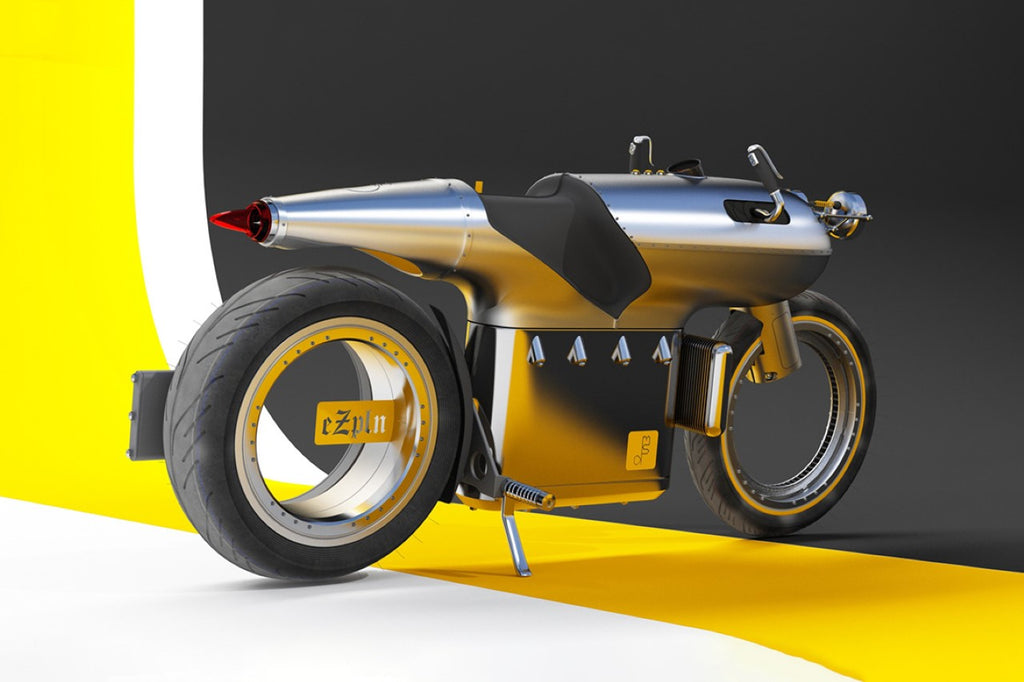The image depicts a futuristic, concept motorcycle that appears to be 3D-generated. The body of the motorcycle resembles an industrial steam tractor, characterized by a singular, metallic column extending forward to a rounded front and tapering to a red point at the rear, likely functioning as a taillight. The embedded seat is set within this column, adorned with rivets that accentuate its industrial aesthetic. The engine area features a chrome, flask-like cartridge inserted into the frame. 

The motorcycle's wheels are black and rimless, presenting a hollow interior; the front wheel shows some form of connection to the frame, while the rear wheel seemingly floats without visible support. The handlebars and headlight are present, and the motorcycle rests on its kickstand.

The backdrop is a striking color gradient, transitioning from white in the bottom left to yellow and then to black, with the motorcycle positioned on the white section and angled toward the black, creating a dramatic effect. The overall setting and design elements convey that this motorcycle is more of a graphic design piece than a functional vehicle.